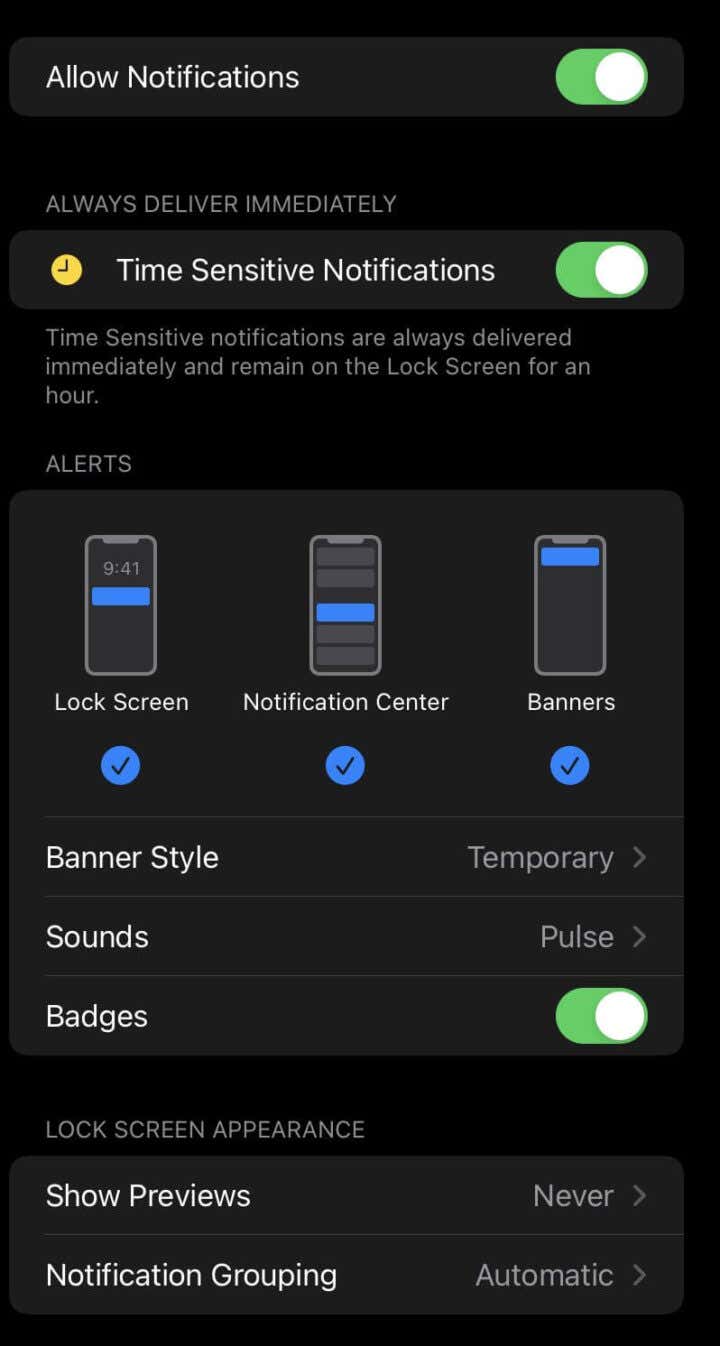This screenshot captures the "Notifications" settings page of an iPhone, set against a black background. At the top of the screen, the "Allow Notifications" toggle is turned on, indicated by a green and white switch. Below, in smaller text, it states "Always Deliver Immediately."

Following that, there's a "Time-Sensitive Notifications" toggle, which is also enabled. The accompanying small text elaborates: "Time-sensitive notifications are always delivered immediately and remain on the lock screen for an hour."

Next, the section labeled "ALERTS" in all-caps features three icons representing different alert delivery options. Each option shows how alerts can be received:
- "Lock Screen" has been selected, highlighted in blue.
- "Notification Center" is also selected.
- "Banners" is again selected.

Further down, the "Banner Style" is set to "Temporary." For notification sounds, "Pulse" has been chosen, and "Badges" are toggled on.

Towards the bottom of the page, the "LOCK SCREEN APPEARANCE" menu item leads to two more settings:
- "Show Previews" is set to "Never."
- "Notification Grouping" is set to "Automatic."